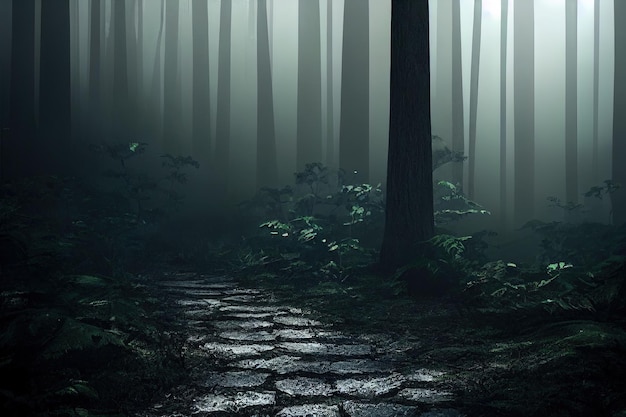The image artistically captures a dense and moody forest scene enveloped in a green haze and mist, suggesting a foggy nighttime ambiance. Tall trees stretch upwards, their long, thin trunks dominating the backdrop, with no branches visible. The forest floor teems with shorter plants, including lush ferns and bushy vegetation, adding depth and texture to the scene. A well-worn, light gray cobblestone pathway curves gently to the left, inviting the viewer to wander deeper into the mysterious, dimly lit forest. The stones of the pathway, aged and weathered, enhance the timeless, enchanting atmosphere of the illustration.